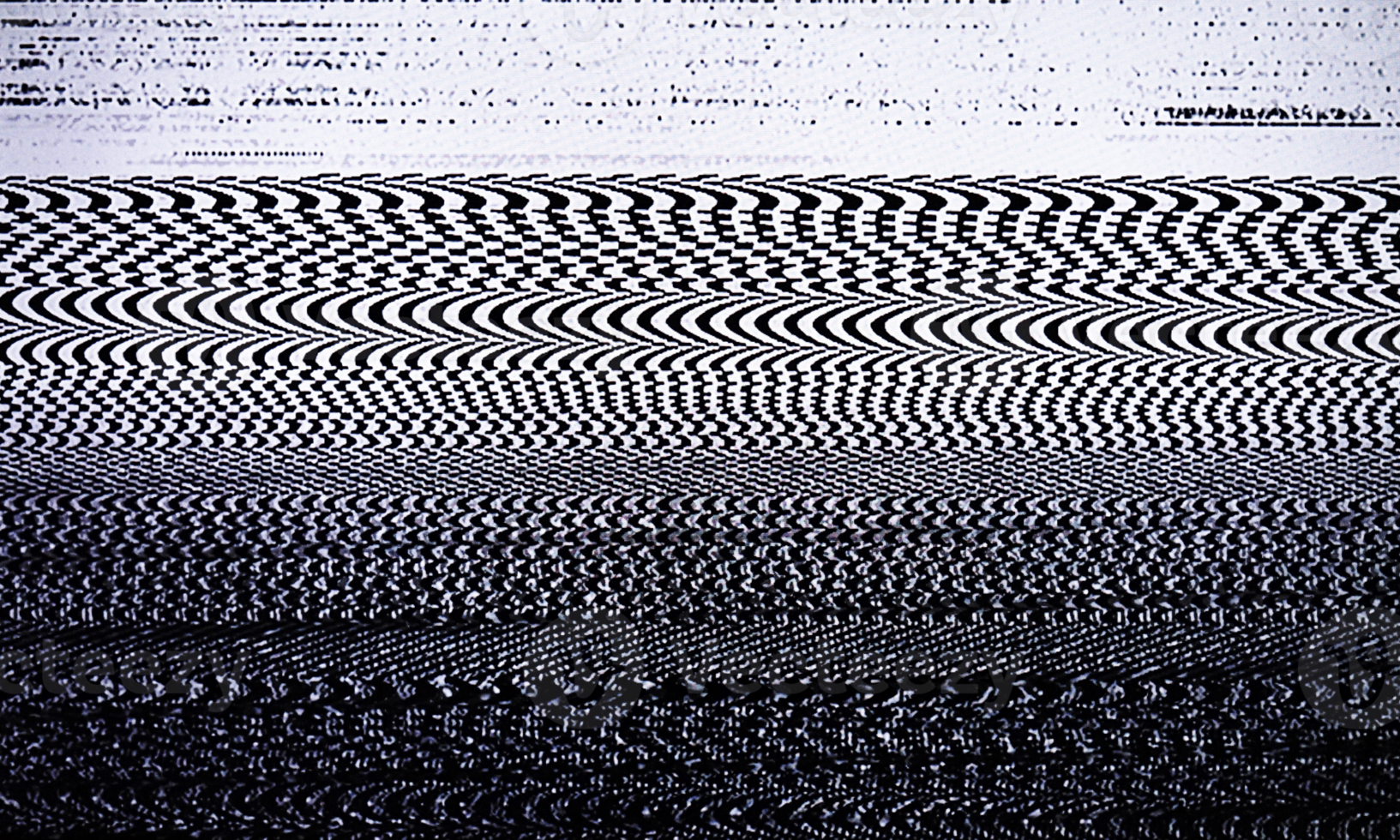The image depicts a classic television static scene reminiscent of rabbit-eared sets from the 50s or 60s. The top portion of the screen is slightly more visible, showing a light gray area with a barely legible logo and text. The logo appears to be a stylized 'G,' and the fragmented word beneath it seems to spell "Vecteezy" although only the bottom halves of the letters are visible. The static is most intense at the bottom, rendering the image progressively more chaotic. The static pattern is divided into distinct horizontal bands with varying designs. Starting at the top, light gray static with scattered black dots forms a line pattern. Further down, the static becomes darker and more complex, transitioning through curvy, almost checkerboard patterns, and into small, darker segments that adopt a herringbone appearance. These patterns create an illusion of movement, akin to the flickering motion of vintage TV static. The lowest portion of the image is dominated by denser, overlapping static that blends into near indistinction between black and white, reminiscent of coarse fabric layers such as denim. The image culminates in an abstract, almost 3D illusion where the patterns appear to shift and overlap as though reacting to the viewer's perspective.